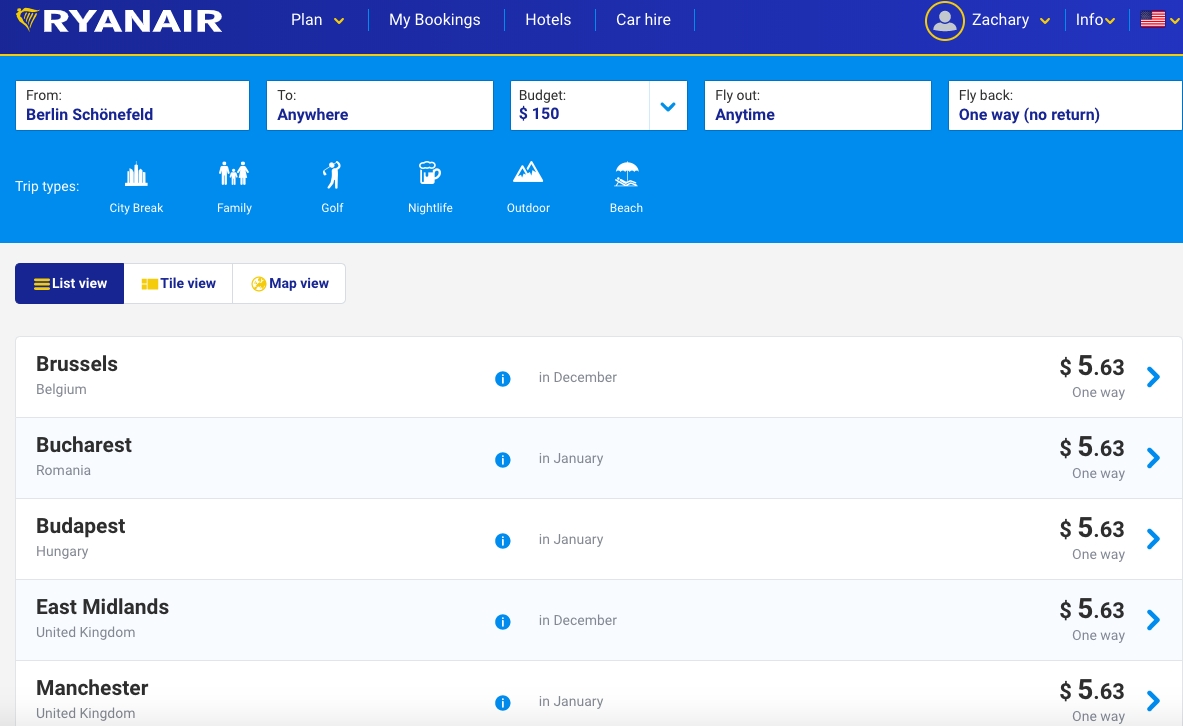The image appears to be a webpage from the Ryanair website, as indicated by the "Ryanair" logo in white text situated at the top left corner. Below the logo, there are several options in a menu bar: "Plan," "My Bookings," "Hotels," and "Car Hire." To the right, there is a yellow circle icon next to a profile labeled "Zachary." Beside this profile information, there are additional icons: an American flag, a simple down arrow, and a larger rectangular blue box.

Within the blue box, there's a search field with flight information that reads "From Berlin Schoenfeld to anywhere." The budget is set at "$1.50," with flexible travel options indicating "Fly out any time," "Fly back one way, no return." The trip types listed include "City Break," "Family," "Golf," "Nightlife," "Outdoor," and "Beach."

Below this search box, several flight options are displayed:
1. **Brussels, Belgium - December:** Priced at $5.63 one way.
2. **Bucharest, Romania - January:** Priced at $5.63 one way.
3. **Budapest, Hungary - January:** Priced at $5.63 one way.
4. **East Midlands, United Kingdom - December:** Priced at $5.63 one way.
5. **Manchester, United Kingdom - January:** Priced at $5.63 one way.

Additionally, there are different view options available for browsing: "Vegas View," "Tile View," and "Map View."